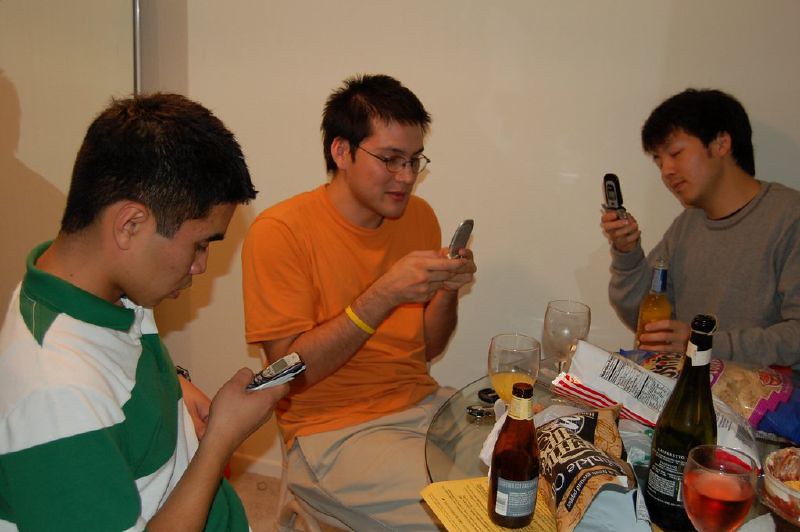In this vibrant, color photograph, three young men of possibly Asian or Hispanic descent are seated around a cluttered, round glass table that features a variety of snacks, including chip bags, and an array of drinks — possibly wine, beer, or juice. Each man is engrossed in an old phone, hinting at a nostalgic or retro vibe. The man on the left, in a white T-shirt with large green stripes, is holding an early 2000s Nokia phone with a distinctive oval shape. The individual in the center, clad in an orange T-shirt and khaki pants, has short hair and glasses, and is using a silver flip phone. On the right, the third man is wearing a long-sleeved gray sweater and is engaging with a black and silver flip phone. Behind them, there is a plain white wall, adding a stark contrast to the lively scene at the table, which suggests a casual, intimate gathering or a small party.